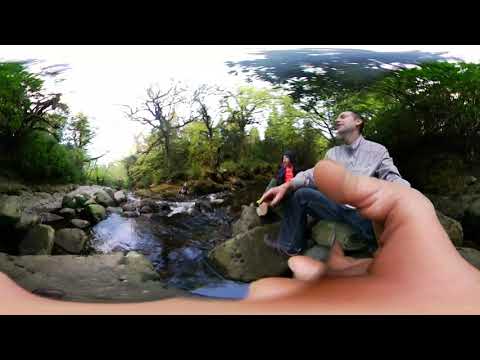In this detailed outdoor image, we observe a tranquil nature scene framed by a black border at the top and bottom. At the heart of the image lies a small body of water—a rivulet with a gentle waterfall cascading from beneath a stone dam. Centered in this picturesque setting is a man dressed in blue jeans, sitting relaxed on a large rock with his head slightly tilted back and eyes closed as if dozing off. Beside him, a thermos is casually placed. In the foreground, a prominent hand with visible thumb and fingers captures attention, seemingly reaching towards the viewer, though its purpose remains unclear. Behind the man, another individual clad in a red shirt and plaid hoodie stands, adding more context to the scene. The background features a few trees, some grass, and the expansive sky visible in the upper left corner, indicating it's daytime. The palette of colors in the image includes tan, gray, pink, blue, black, orange, light green, and a touch of brown, contributing to the natural, serene ambiance of this moment captured in nature.